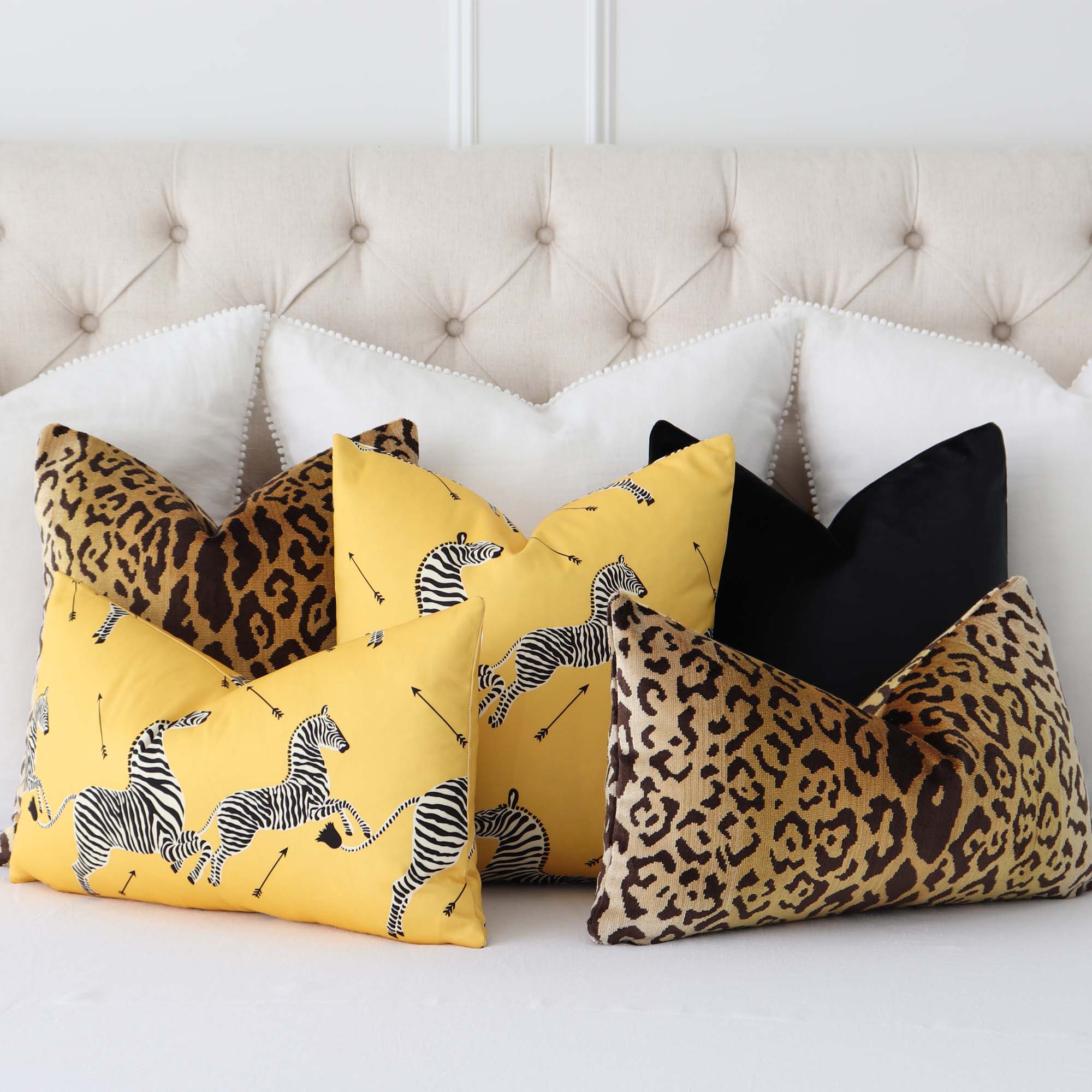This square color photograph features the upper section of what appears to be a bed or a daybed, set against a white wall. A white or off-white headboard spans the width of the image, partially obscured by an array of throw pillows. Three prominent white pillows form a backdrop, with the central pillow extending slightly higher and displaying a subtle V-shaped top. Adorning the foreground are diverse, vibrant pillows: a leopard print pillow on the left and a black pillow on the right, both sporting similar V-indents at their tops. Nestled between these are two yellow square pillows, each embellished with zebra illustrations and small arrows. Additionally, a thinner, rectangular yellow pillow with zebras overlaps slightly in front of the leopard print pillow. The composition is completed with another rectangle-shaped leopard print pillow to the right, featuring the characteristic V-top pattern and blending harmoniously with the white sheet or blanket that covers the bed. This setting exudes a sophisticated yet eclectic style, possibly indicative of a hotel room ambiance.